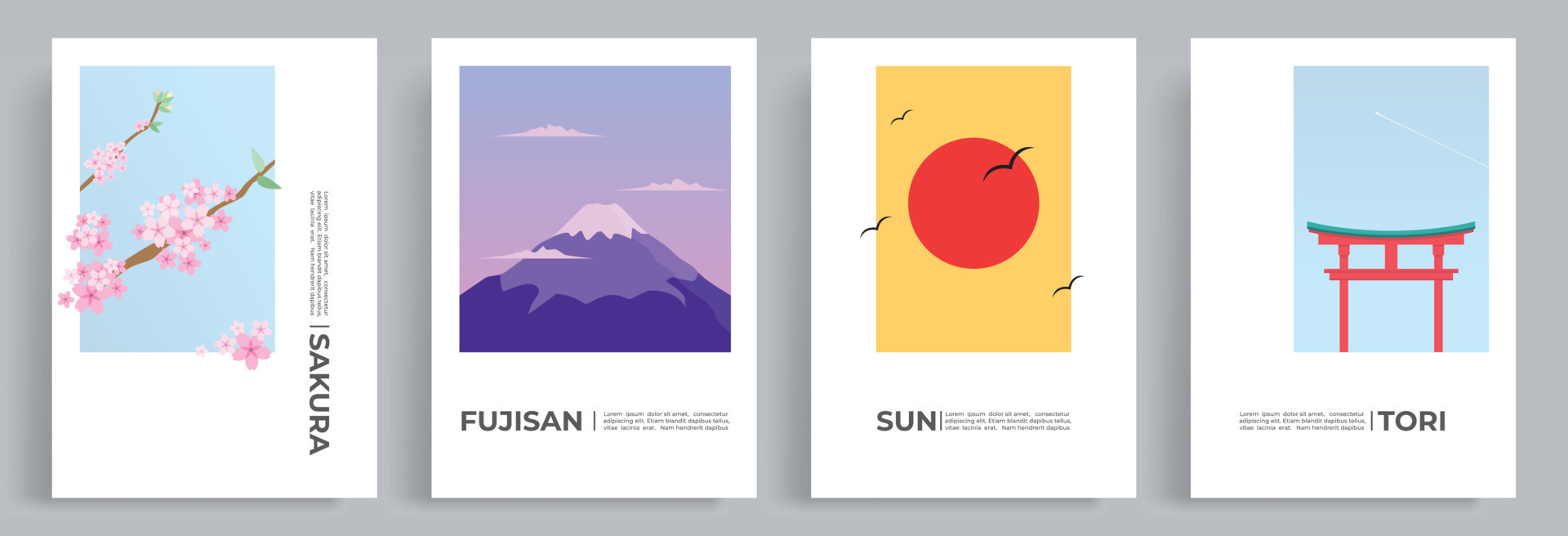The image features four distinct art pieces set against a dark gray background. Each piece has a shared white backdrop. On the far left, pink cherry blossoms extend beyond the borders of a vertical blue rectangle, accompanied by the word "SAKURA" running vertically alongside. To its right, a piece showcases a majestic, snow-capped mountain under purple skies, captioned "FUJISAN" with a gradient of light to dark purples and white clouds. The third piece from the left depicts a bright orange sun set within a yellow rectangle, with four birds in flight below the word "SUN." The final artwork on the far right features an architectural structure resembling a temple with a stylized blue roof and orange framework, labeled "TORII" underneath.